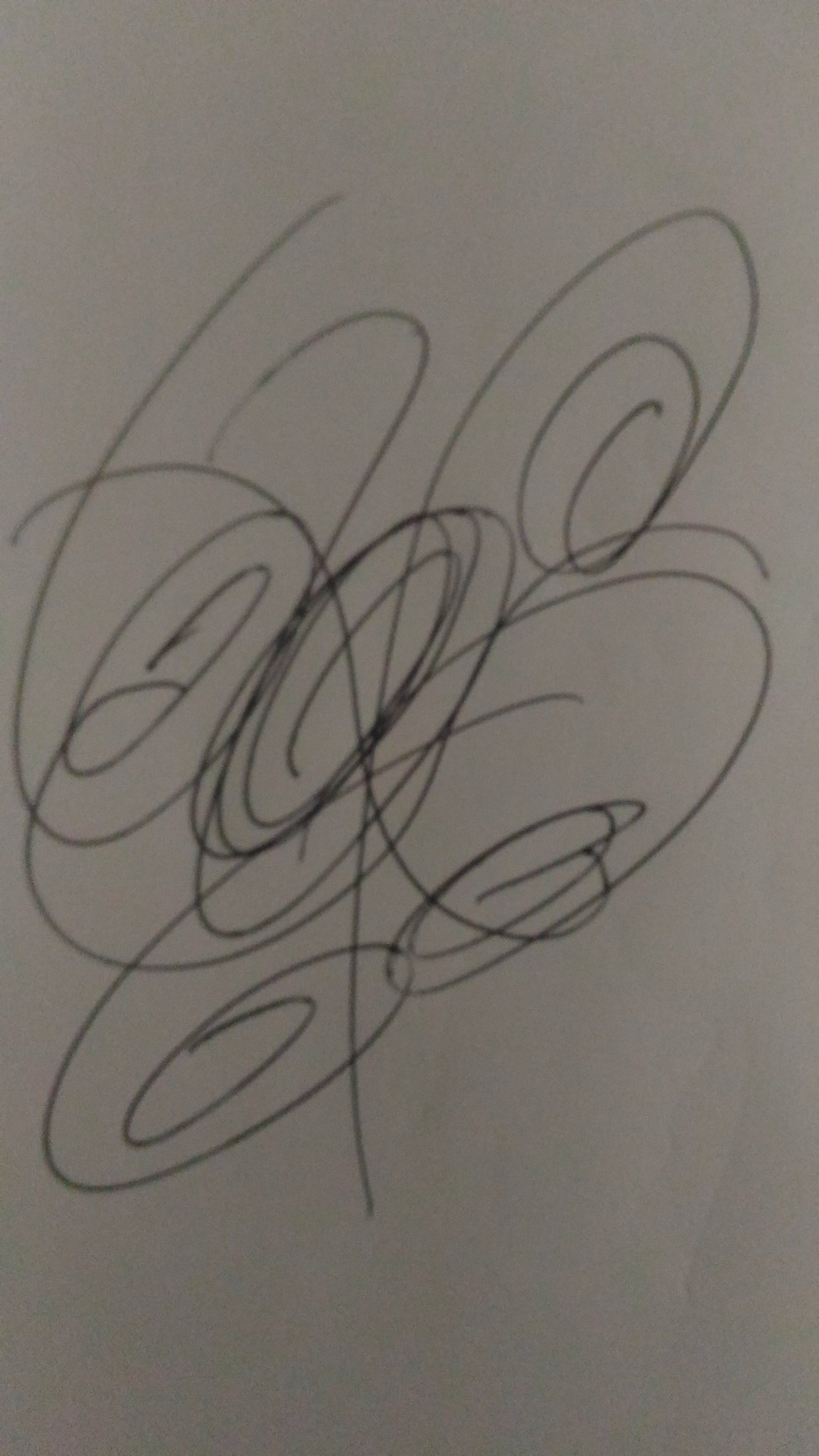A pen drawing on a plain sheet of white paper features an intricate labyrinth of continuous swirling lines that appear predominantly concentrated in the center. The central swirl is the largest, dominating the composition. Extending outwards, similar swirling patterns are located in roughly four corner regions, each seemingly initiated without lifting the pen from the paper. The swirls converge and diverge, creating an almost hypnotic effect, and the connections between these sections blur the beginning and end points of individual lines. The white paper shows faint creases, suggesting it may have been folded or pressed against another surface. There are also faint, indistinct lines visible on the reverse side, hinting at an additional layer of random sketches that do not overshadow the main swirl design.